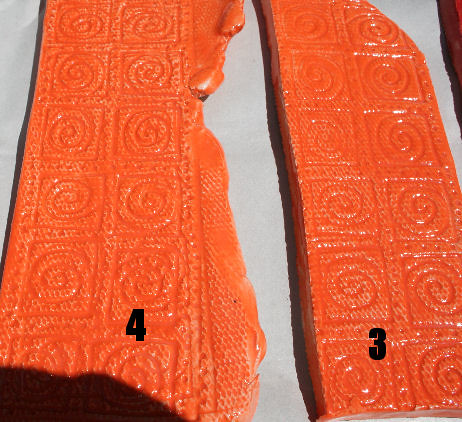In an outdoor setting, this photograph showcases two decorative orange slabs, likely made of marble or stone, with intricate, indented swirly designs. The slabs are unevenly shaped and are laid out vertically next to each other on a white background, possibly a piece of paper or fabric. Both slabs exhibit a sequence of square patterns with swirly circles inside them, arranged in rows of two and columns of six, separated by small dots to add texture. On the left slab, the number "4" is prominently displayed in black, and on the right slab, the number "3" is similarly marked. A faint shadow, presumably of the photographer, is visible in the bottom left corner of the image.